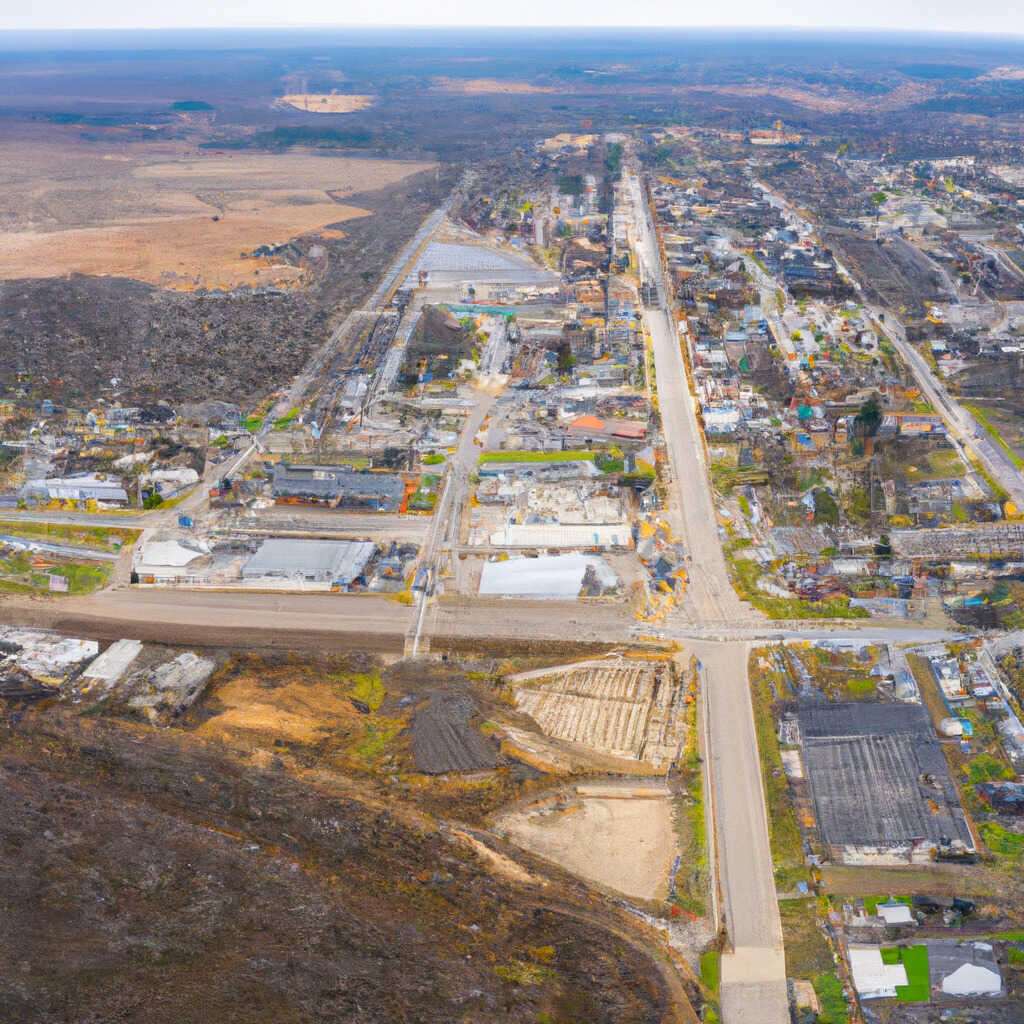This aerial photograph captures a detailed view of a semi-developed area that blends industrial, suburban, and undeveloped landscapes. Taken from a high vantage point, possibly a drone or an airplane, the image reveals an intricate tapestry of human development and natural land. To the left, there's a barren, desert-like expanse with minimal vegetation, characterized by tan-colored sand and dirt, suggesting future development potential. This barren land wraps around the top of the photograph, giving way to rolling hills and a distant horizon that fades into a soft blue.

In the center and towards the right side of the image, a more developed suburban or industrial area is visible. This section is marked by numerous buildings, homes, and factories, interspersed with open fields. The streets are dominated by a palette of brown, green, gray, and cream, with major roads standing out as thick lines compared to thinner minor roads. Some green vegetation and trees are scattered throughout this urban patch, providing contrast to the otherwise brown and gray tones. Parking lots, shopping centers, and possible downtown areas contribute to the complexity of this developed land. The overall flat terrain, with slight undulations, supports the realistic and highly detailed representation of this region.